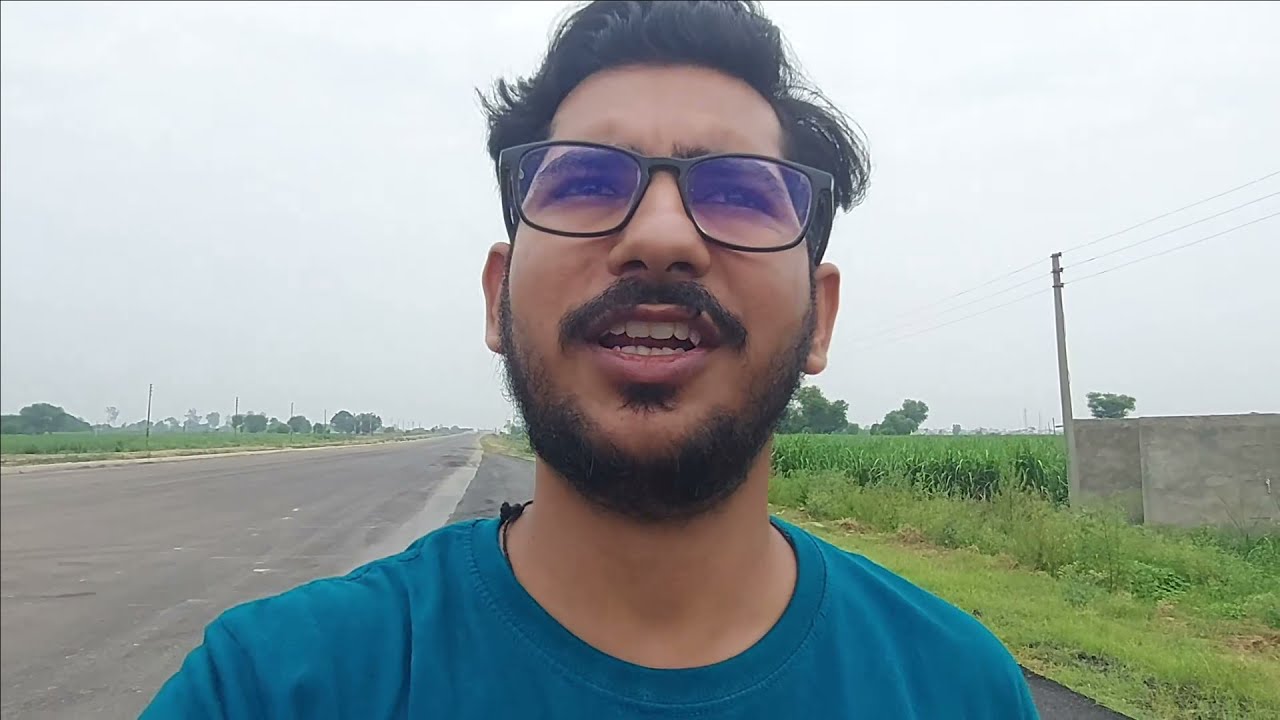The image captures a selfie of an Indian man standing outdoors in a rural area near a road. The man, wearing a turquoise blue t-shirt with a cord necklace partially visible, has short black hair parted to the side, and is sporting black-framed glasses. He also has facial hair consisting of a mustache, beard stubble, and a patch beneath his lower lip. He appears to be mid-sentence, looking upwards with his mouth open, possibly recording a video. Behind him, the scene features a hazy, overcast sky and a mix of green grass, tall shrubs, and trees along both sides of the asphalt road. Telephone poles and wires line the road, which stretches into the horizon. Additionally, there are two gray cement structures near the crops, which seem to be corn, adding to the rural setting. The man is positioned off to the side of the road, and the photo frame captures him from the top of his head to just below his shoulders.